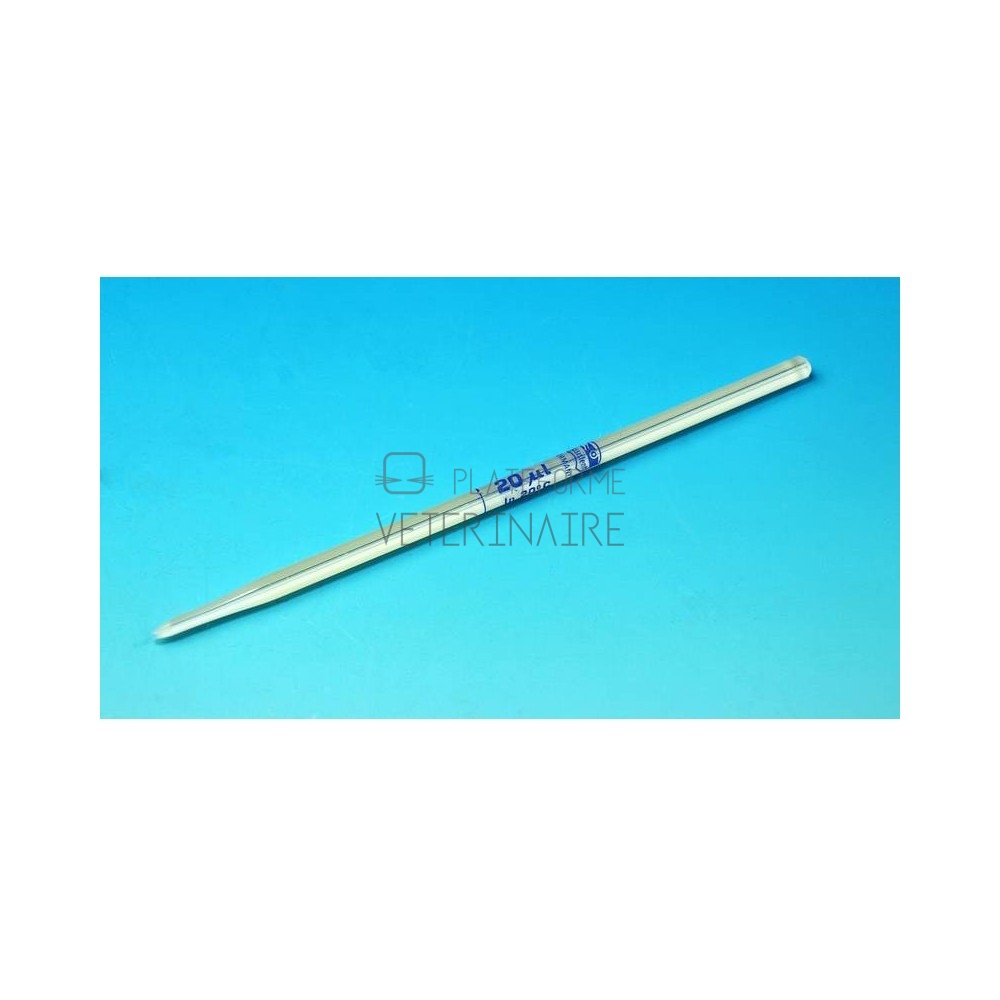In the image, a long silver object, resembling a pipette or specialized pen, diagonally spans a light blue background from the top right to the bottom left. The object appears almost translucent with a white and gray hue, giving it a glass-like impression. Written on the pipette are blue letters that read "20 ML N20SC" and "PLA... RME," with "VETERINAIRE" prominently stamped across its center. Above this stamp, there's a small square box with whisker-like lines extending from it. The setting is minimalistic, emphasizing the object in the center of the rectangular blue area.